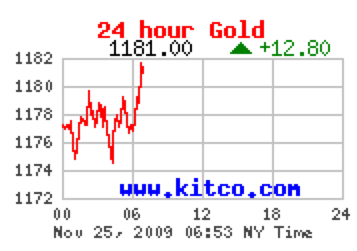The image is a small horizontal rectangular screenshot tracking the 24-hour gold price on November 25, 2009. Displayed prominently at the top in red is "24 hour gold" followed by the figure "1181.00." Underneath, a green triangle points upwards, accompanied by text indicating a rise of "+12.80." The graph itself is rendered in vibrant red, showing a steady line at first that then climbs sharply. The vertical price range spans from 1172 to 1182, with the red line starting around 1177 and fluctuating before reaching the peak at 1181. The x-axis denotes time with markings at 0, 6, 12, 18, and 24 hours, aligning with the timeline labeled in New York time. At the bottom, the date is clearly marked, and the blue text of the website "www.kitco.com" provides the source.